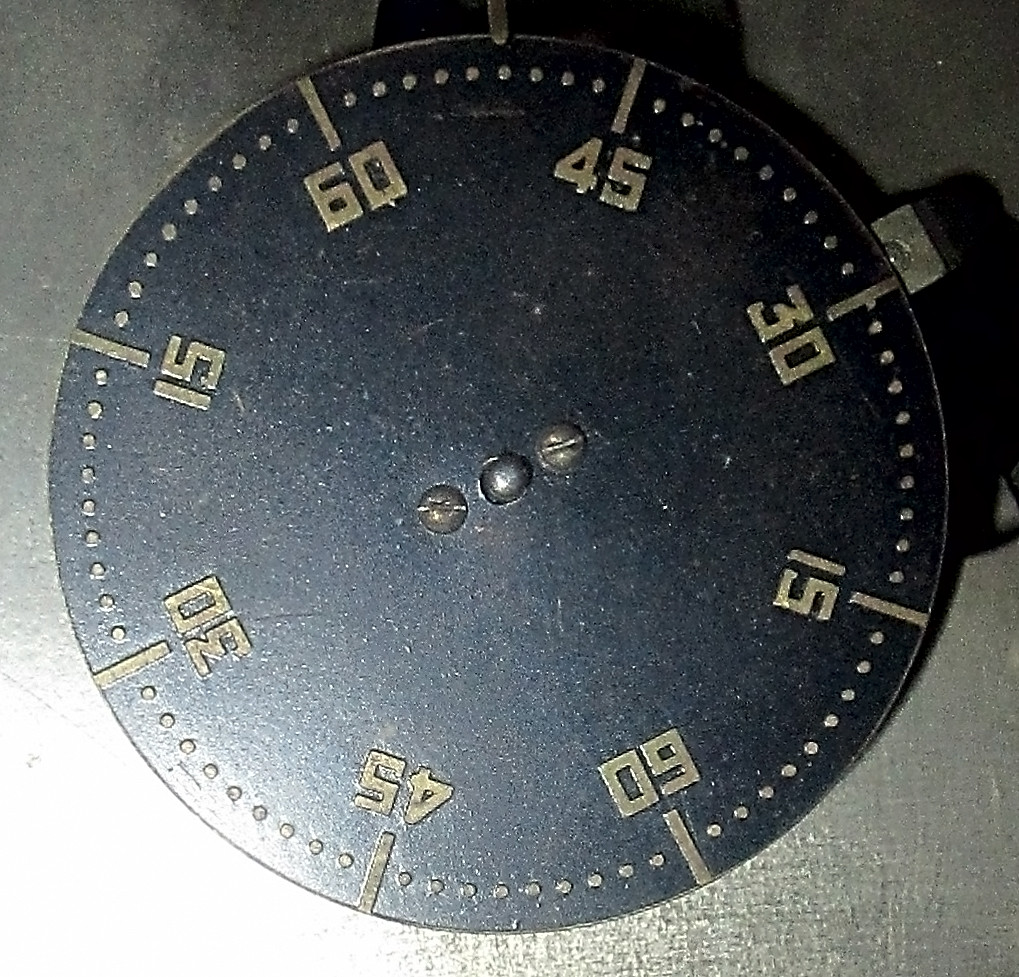This image depicts an old, round timer or clock with a black face, possibly made of metal, plastic, or flakeboard, featuring gold numerals marking 15-minute intervals—45, 30, 15, 60—arranged repeatedly around the edge. Silver studs accentuate the circumference, with gold dots distributed between the numerals. At the very top, a protruding piece indicates the time. In the center, a thick silver screw secures the device to its base, flanked by two flathead screws. The background of the image is a light gray or grayish-black color, with the bottom left notably illuminated, casting a white light. The clock's function appears unclear as it isn't seemingly operating.